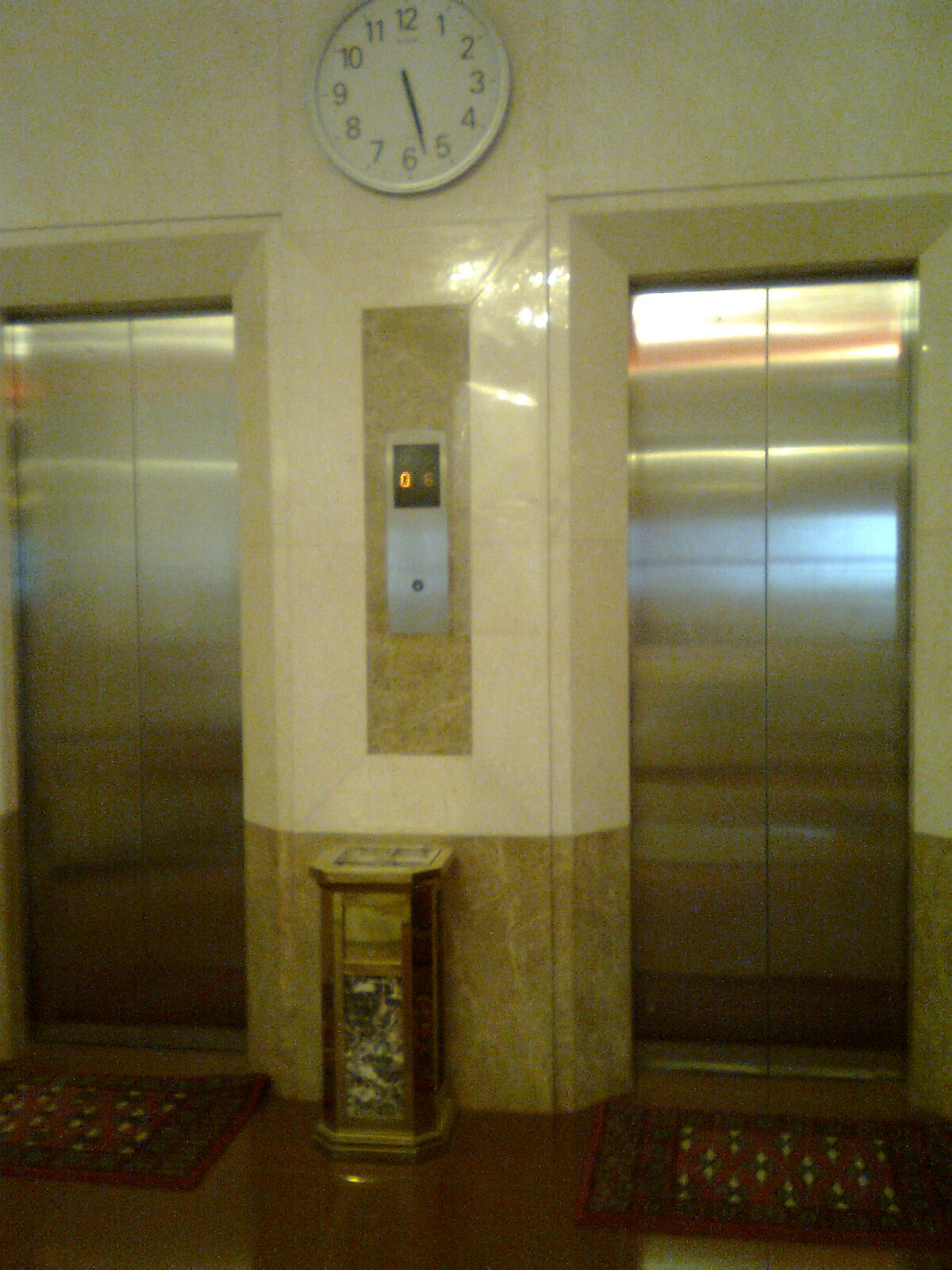This image depicts the interior of a sophisticated building, likely an office or hotel, focusing on two closed, narrow, silver elevators positioned side by side. The scenario presents a polished and somewhat opulent setting, with a wall behind the elevators exhibiting a marbled appearance in white and yellow tones, accented by brown streaks. Between the elevators, a digital display indicates the floors the elevators are on, and directly above this display is a white round wall clock showing the time as nearly 6:30. Below the display, there's a square object that could be a garbage can or an ashtray resting against the wall. At the base of the elevators, there are two welcoming red carpets adorned with blue and white spots, laid out on a glossy, potentially marble floor that gleams under the building's lighting.